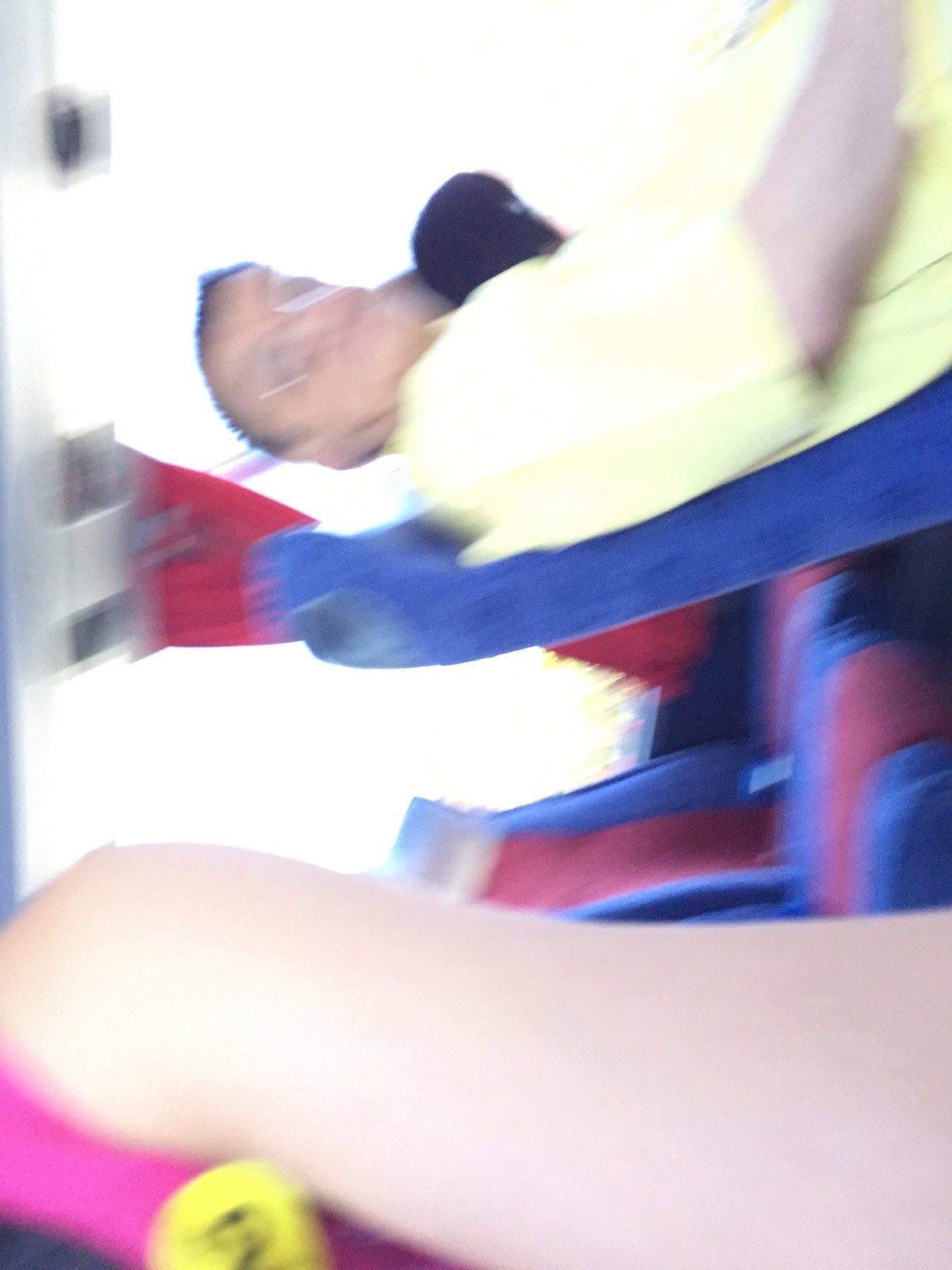The image is a very low-quality and blurry, sideways photograph taken inside a commuter or passenger bus. The camera is turned back towards the person taking the picture, whose arm is visible in the lower part of the photo, wearing a deep pink shirt with a small yellow button. The upper part of the photo shows a young person with short hair and glasses, sitting in a blue seat and wearing a light yellow shirt and possibly a white hat. The bus seats are partly visible behind this person, with a distinctive color pattern: the sides of the seats are blue and the centers are red. There is also a large white glare near the bottom of the image, possibly another seat, and what looks like a gray overhead compartment with two black squares at the top of the picture. Overall, the image is difficult to discern clearly due to its blurriness and sideways orientation.